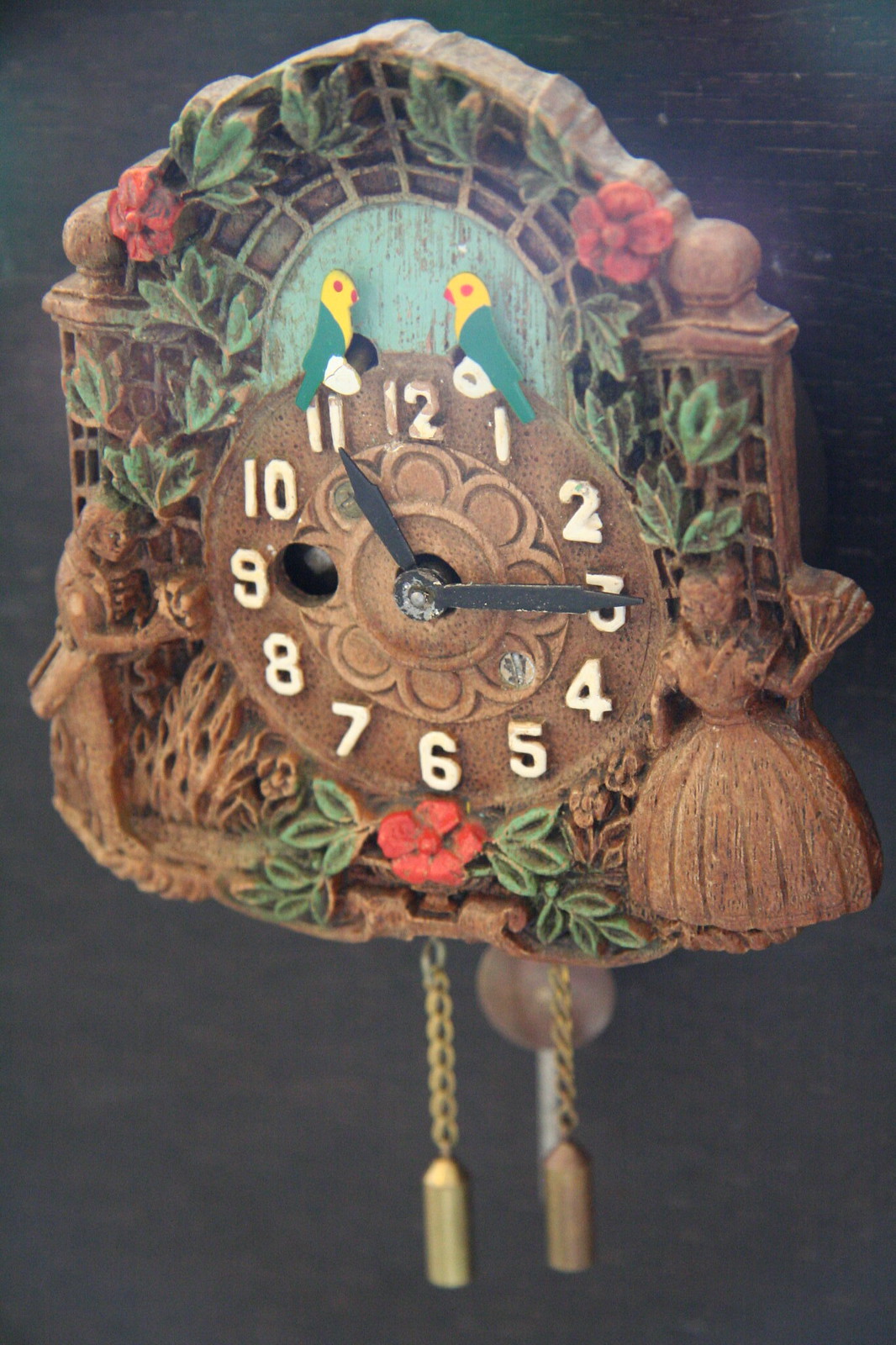This detailed photograph captures a beautifully intricate old-fashioned cuckoo clock. Carved from dark-colored wood, the clock features a three-dimensional texture enriched with numerous carvings and castings, highlighting its meticulous craftsmanship. The clock face displays white painted, raised numbers—though the number 12 shows signs of wear, tinged with brown. The black hour hand is set at the 11, and the minute hand points to the 3, indicating the time is quarter past 11.

Above the clock face, two colorful parrots with green feathers, yellow heads, and red eyes and beaks perch on a rod, facing each other. An arch painted pale blue frames them, adorned with additional green leaves and red blooms. Flanking the clock face are carvings of a man and a woman. The man, dressed in an old-fashioned tailcoat and breeches, holds a bouquet of flowers extended outward. The woman wears a long, full-skirted dress and appears to be holding a fan in her left hand, looking towards the man. Surrounding these figures are non-painted carvings of plants, grasses, and flowers.

Below the clock face, a red flower with green leaves stands out. The lower section of the clock features a bronze pendulum shaped like a small circle, flanked by two brass chains with golden weights resembling tall candles, which likely function as mechanisms for adjusting the clock. The intricate designs also include pillars with rectangular inset patterns, topped by rounded finials, encapsulating the rich detail that makes this cuckoo clock a stunning piece of craftsmanship.